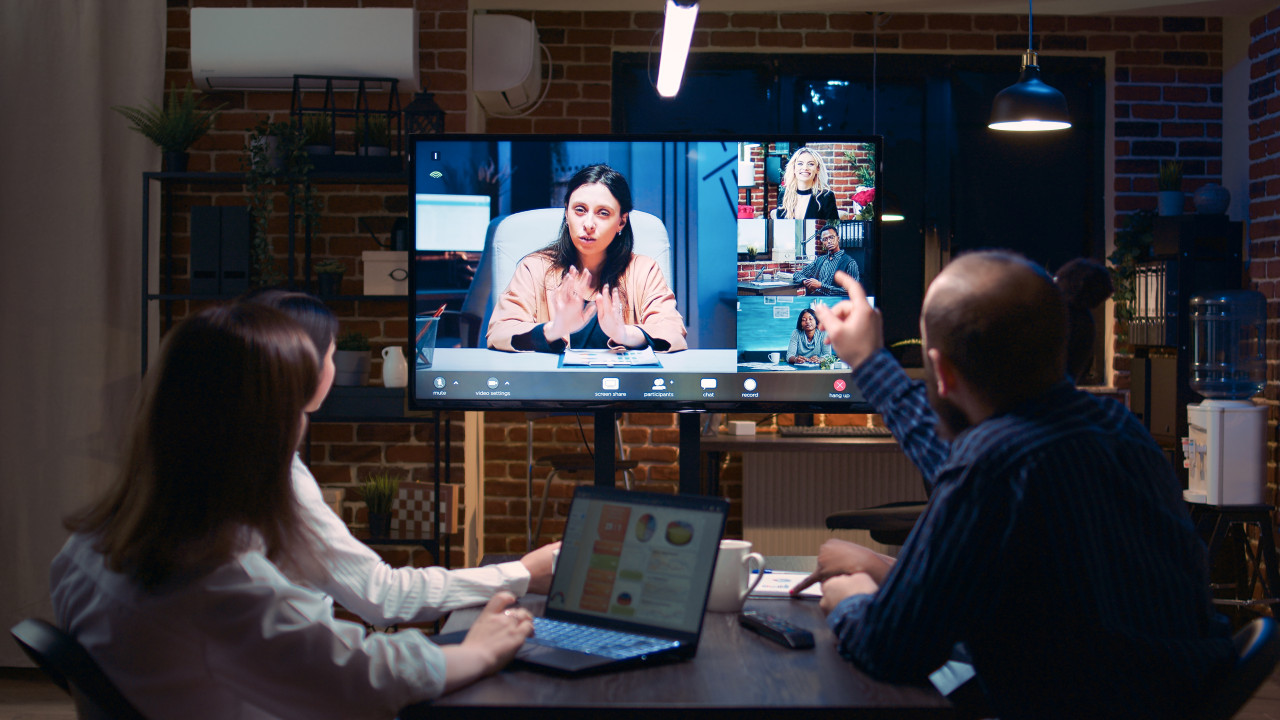In the image, a group of people gather around a coffee table, engrossed in a video conference displayed on a large monitor. Seated at the coffee table's right side is a balding man with a beard, dressed in a blue and navy striped shirt, gesturing towards the screen. On the left side of the table, two women in white dress shirts focus attentively, one with an open laptop in front of her displaying a menu. The primary monitor showcases a woman with long black hair and a brown shirt speaking animatedly from an office chair. Beside her, three smaller video feeds feature other participants: a blonde woman with long hair, an African-American man, and an Indian woman. The backdrop of this meeting room consists of a red brick wall adorned with a blue metal-framed bookcase stocked with various blue items, white cups, and vases. To the right, a white water cooler with a blue tub stands, enhancing the office ambiance. Above, a fluorescent lamp and a bullet lamp hang, illuminating the scene of this modern collaborative workspace.